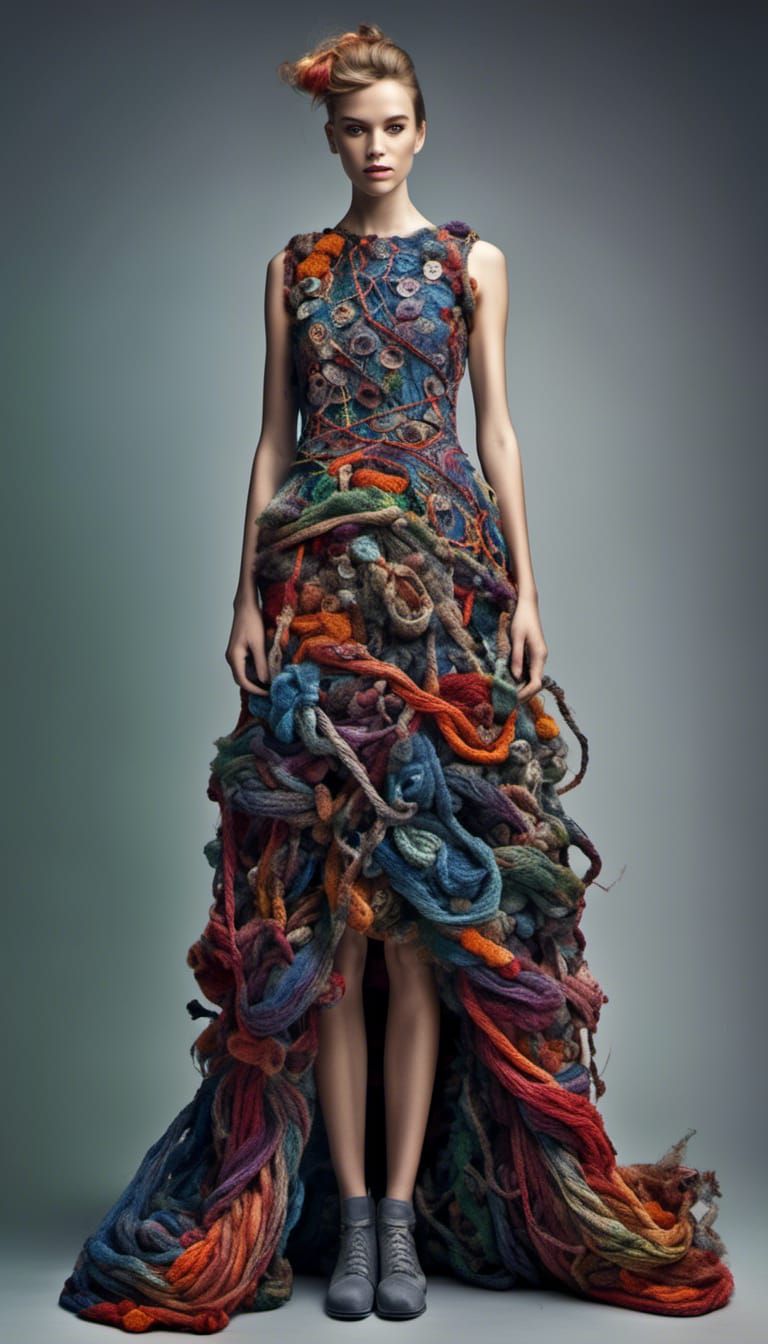The image features a towering model with her brown hair neatly pulled up into a bun, modeling an intricate and unique dress. The dress appears to be AI-generated or photorealistically illustrated, suggesting an artistic flair. It is sleeveless with a high neckline and fits tightly against the model's torso before flaring out into an almost A-line shape past her natural waist. The fabric of the dress is composed of what seems like haphazardly assembled, braided ropes and rolls of yarn in various muted but still colorful tones, including blues, purples, reds, oranges, greens, and grays. These colorful threads create an abstract, textured design all the way down to the floor, although the front hem is higher, exposing her knees and calves. The model completes the look with gray lace-up boots that reach her ankles, enhancing the avant-garde style of the ensemble.